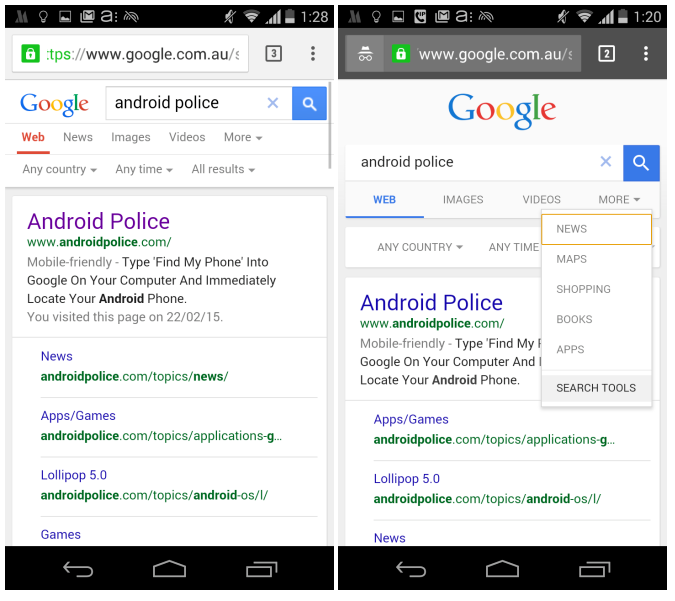The image consists of two side-by-side screenshots showcasing someone using Google Search to look up "Android Place." Both searches are conducted on the Australian version of Google, likely from a smartphone or portable device given the small and compact screen sizes.

In the first screenshot, the search results prominently display "Android Place" as the top result, followed by related news articles, apps, and games, with mentions of Lollipop 5.0 towards the bottom. Contrastingly, the second screenshot shows a slightly different order: "Android Place" remains the first result, but it's followed by apps, games, lollipops, and news articles.

Notably, the second screen appears to be zoomed in, making the Google logo more prominent and pushing the search results further down, which reduces the number of visible results. This subtle difference highlights the variability in search result display, despite being conducted from the same geographical location – Australia.